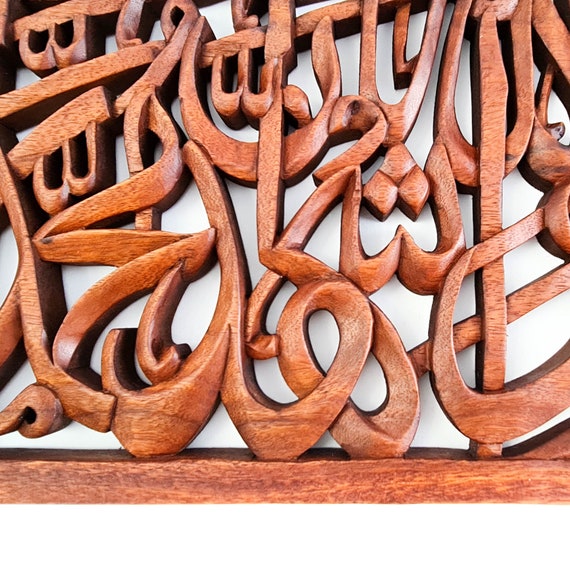This is a photograph of an intricate wood sculpture set against a plain white background. The sculpture, which has an orangey-brown or medium brown, almost cherry-like hue, features a wood grain pattern and appears to be expertly sanded down to a smooth finish. The piece is composed of various elaborate, curvy shapes including spirals, squiggles, and diamonds, forming a complex and aesthetically pleasing arrangement that suggests influences from exotic or foreign scripts, potentially resembling Asian or Arabic alphabets. The wood shapes seem to integrate into one another in a smooth, flowing manner, creating an impression of letters or symbols snaking around each other. Shadows within the sculpture highlight its depth and thickness. The sculpture appears as if it could be an ornamental piece in a house or an artwork on display, although the exact context remains unclear due to the close framing of the photograph that cuts off the artwork on the sides and top.